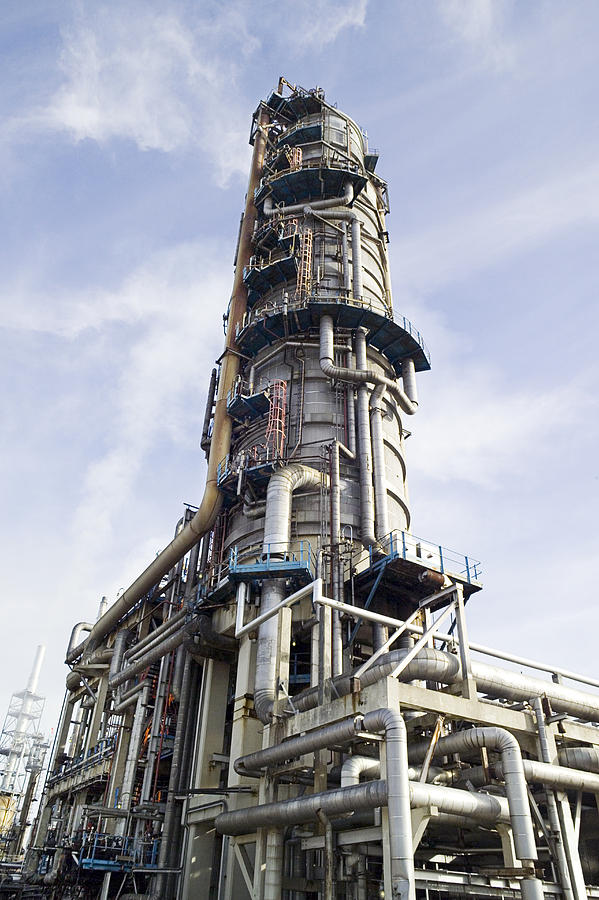The image depicts a highly elaborate and towering industrial structure, likely an oil refinery, characterized by its extensive network of pipes and mechanical components. The central structure, primarily silver or steel in color with occasional bronze, pink, or yellow accents on the ladders, and hints of blue platforms, ascends dramatically into the clear blue sky, which is tinged with slight purple hues and scattered with light, white clouds. Captured from a low angle, emphasizing its towering height and intricate design, the structure is surrounded by numerous pipes and connector pieces extending in multiple directions, adding to its complex, almost skeletal appearance. The industrial feel of the scene is unmistakable, exuding a sense of towering, mechanical grandeur against the serene sky.